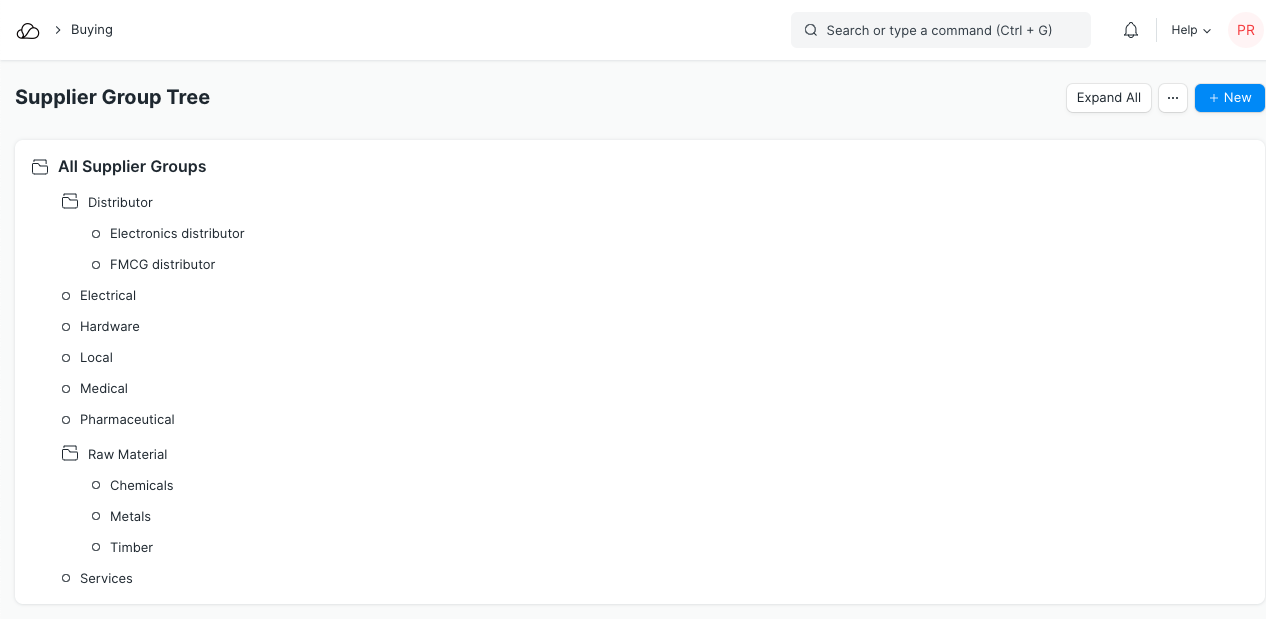The image features a white background with structured elements primarily in black and orange text. In the top-left corner, the word "buying" is prominently displayed. On the top-right, there is a search bar inviting users to "search or type command CTRL + G," accompanied by a bell-shaped notification icon, a drop-down menu labeled "help," and a profile icon displaying the letters "PR" in orange.

The left side of the image is occupied by a hierarchical menu titled "Supply Group Tree." This menu lists a main folder named "All Supplier Groups," which branches into the sub-folder "Distribute." Within "Distribute," further sub-folders include "Electronic Distributor," "FMCG Distributor," and additional categories such as "Electrical," "Hardware," "Local," "Medical," and "Pharmaceutical." Another main sub-folder under "All Supplier Groups" is "Raw Material," which contains the sub-categories "Chemicals," "Metal," and "Tin." Below all these folders, there is an additional section labeled "Services."

In the top-right part of the image, three distinct buttons are visible. The first is a blue "Add" button, featuring white text that reads "Brand New," indicating the option to add another supplier group. The other two buttons are white with black text, labeled "Expand All" and "Menu".

Overall, the interface is clean and user-friendly with a clear white background enhancing the readability of the menu and icons.